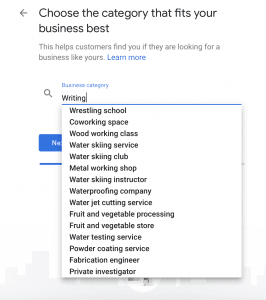A voice-formulated image description has been cleaned up and transformed into a detailed caption:

"At the top of the image, there's text advising users to 'Choose the category that fits your business best,' with an arrow pointing to the left. Beneath this guidance, there's a reminder reading, 'This helps customers find you if they’re looking for a business like yours.' Additionally, a blue hyperlink labeled 'Learn More' is present. Below these instructions, the image shows a 'Business Category' section with a text box containing the word 'writing.' The text box features a drop-down menu that lists various options, including 'Wrestling School,' 'Co-working Space,' 'Woodworking Class,' 'Water Skiing Service,' 'Water Skiing Club,' 'Metal Working Shop,' 'Water Skiing Instructor,' 'Waterproofing Company,' 'Water Jet Cutting Service,' 'Fruit and Vegetable Processing,' 'Fruit and Vegetable Store,' 'Water Testing Service,' 'Powder Coating Service,' 'Fabrication Engineer,' and 'Private Investigator.' Another notable element is a blue button labeled 'Next,' situated behind the drop-down menu. There's also a blue line underneath this section. The bottom of the image reveals a faint background of indistinguishable buildings."